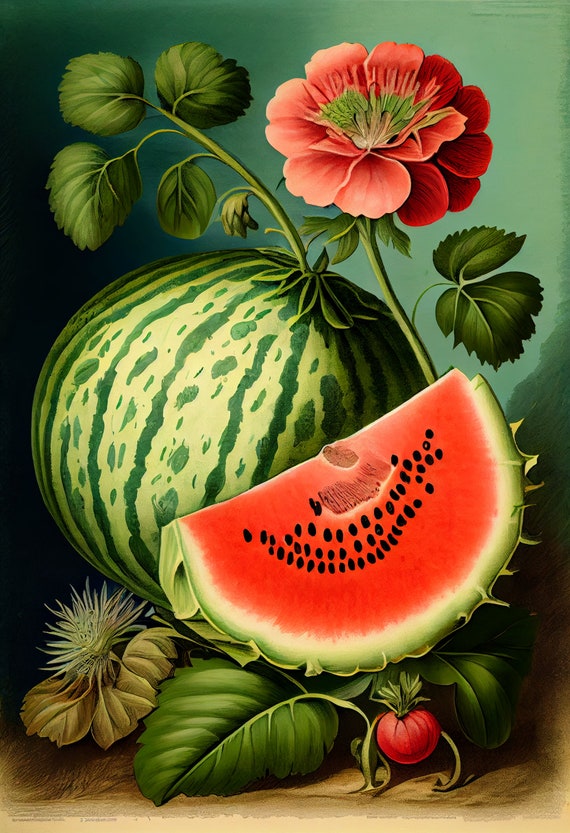This vibrant and highly detailed painting captures the essence of a watermelon plant with stunning accuracy, reminiscent of natural sciences sketches from Victorian-era natural history books. In the foreground, a large wedge of sliced watermelon reveals its bright pink-red interior dotted with black seeds. Just behind it, a whole, uncut watermelon displays its characteristic light green skin with dark green stripes. The green plant, with its intricate network of vines, supports the watermelon and is adorned with lush leaves. Above the watermelon, a striking red flower blooms, its petals radiating from a green center with small blossoms, blending into lighter pinkish-red hues toward the middle. Below, a mix of healthy and dead leaves can be seen, adding depth and realism to the composition. The bottom of the painting features a brown surface, while the background transitions from a shadowy dark green on the left to a softer light green on the right, creating an ombre effect that enhances the overall vividness.